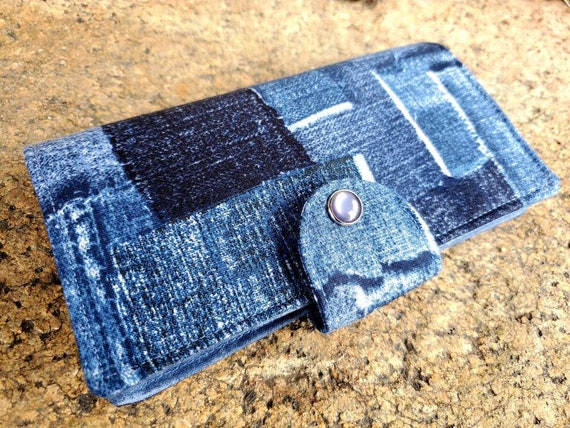This image features a ladies' long wallet made of various shades of blue denim, prominently displayed on a background that appears to be a mixture of tan cork and granite-like materials in different shades of brown and beige. The wallet has a flap that folds over and secures with a silver snap button. The front of the wallet showcases a patchwork design: a medium blue denim pocket with black vertical lines and white edging, a larger dark blue denim section with additional white edges, and a lighter blue denim piece that forms the outermost layer. The wallet lies flat in the center of the photograph, and its detailed stitching and the distinct texture of the denim make it a visually appealing accessory.